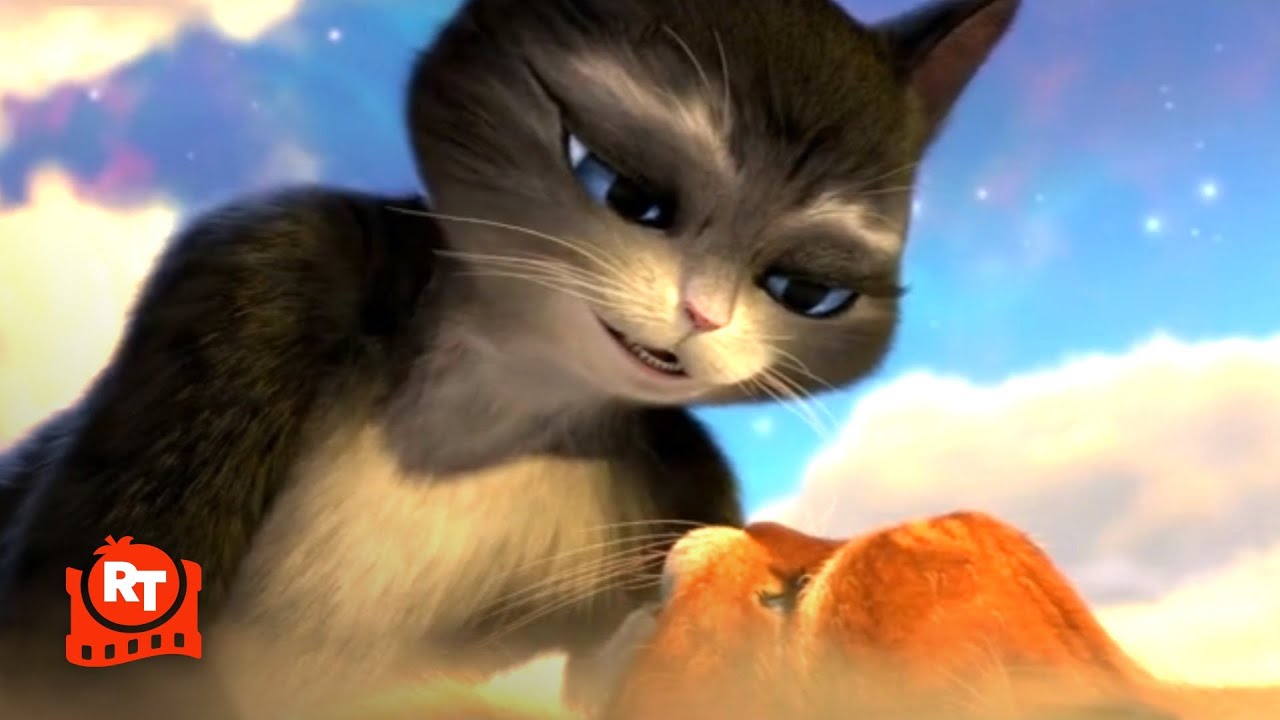This image appears to be a still from an animated movie or television show featuring anthropomorphic cats set against a vivid, celestial backdrop. The scene is framed by a bright blue sky adorned with sparkly stars and large, fluffy white clouds, giving the impression that the characters are high up in the sky. Two feline characters dominate the image; the larger cat—characterized by dark greyish-black fur, striking blue eyes, beige chest fur, and human-like facial expressions—looms over another cat. This second cat, lying on its back and gazing upwards, sports reddish-orange fur with distinctive white patches around its nose and forehead. In the bottom left corner, there is a notable logo: the letters "RT" enclosed within a black circle, overlaid on a red film strip, indicative perhaps of the production company behind the animation. Prominent whiskers and detailed eyebrow hairs emphasize the expressiveness of both characters.